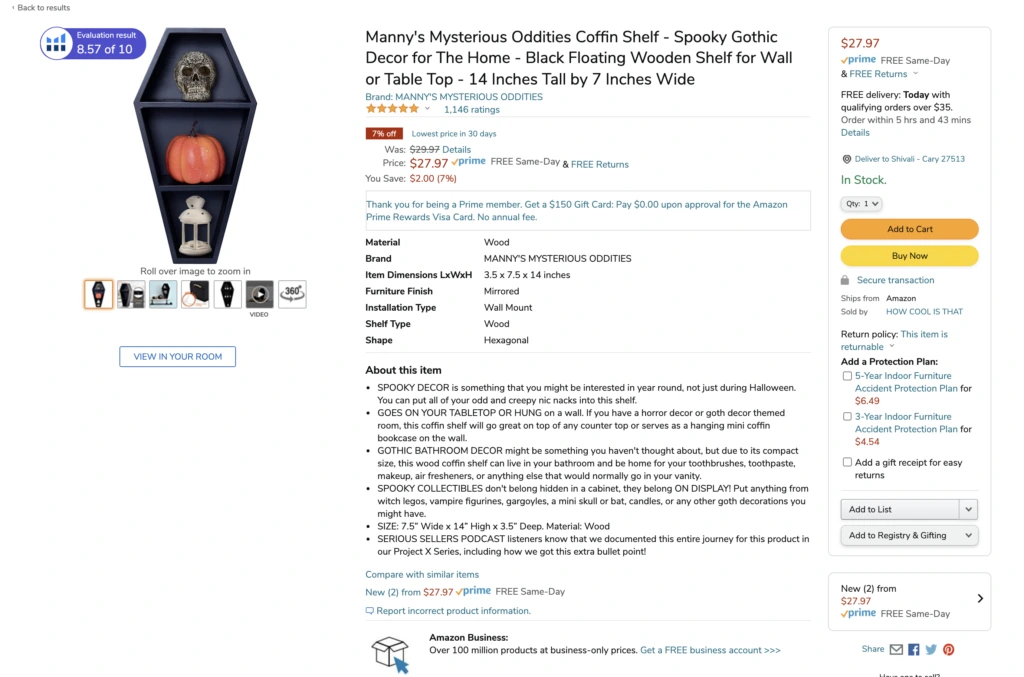This is a descriptive caption for a product image of a unique home decor item on Amazon:

---

A screenshot of an Amazon product page showcasing "Manny's Mysterious Oddities Coffin Shelf." This striking piece of spooky, gothic decor is designed to resemble a stand-up coffin with storage spaces ideal for displaying skulls, pumpkins, and other macabre items. The black floating wooden shelf measures 14 inches tall by 7 inches wide, making it a compact yet eye-catching addition to any wall or table. Listed at $27.97, with a $2 discount available and free delivery for Prime members, the item can be added to your cart or purchased immediately with the prominent "Buy Now" option. The coffin shelf is described as having a wood finish, with mirrored installation types available and a hexagonal shelf shape. Additional purchasing options include protection plans priced at $6 or $4, and there is a return policy in place. This distinctive shelf, sold by Manny's Mysterious Oddities, is currently in stock and ready to bring a touch of eerie charm to your home.